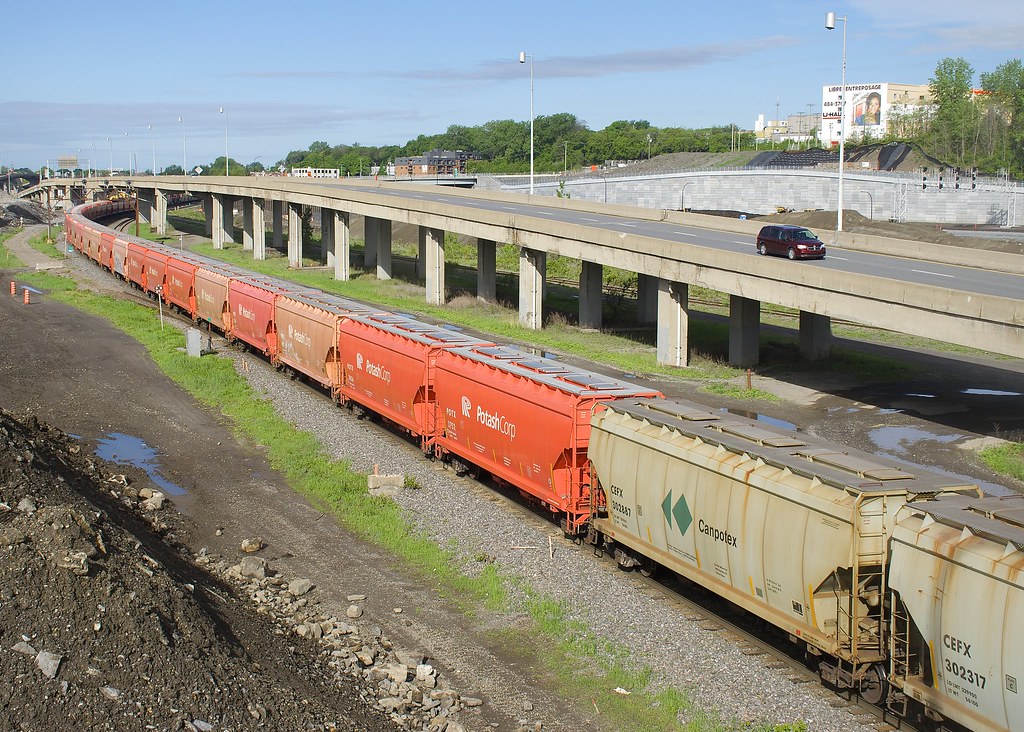The photograph features a long line of railroad cars extending from the bottom right corner, running parallel to a highway. The cars' colors vary from light gray to orange, with one notable light gold car, and are marred with rust stains and darker gray sections on top. The foremost car on the right is marked with a green diamond and arrow emblem, reading "Campo Tex."

To the right of the tracks, a highway bridge spans the railroad, with a single light purple minivan crossing it. The bridge is substantial in length and casts a shadow over the train below. Left of the tracks, a dark brown pile of dirt and a mud puddle are visible, contributing to the industrial landscape.

In the background, beyond the bridge, various structures and roads are discernible, including an additional road area, buildings, and several billboards. Off to the top-right, a cluster of trees and more roadways enrich the scene. The top of the photograph is adorned with a blue sky, streaked with thin wispy clouds, adding a serene backdrop to the bustling activity below.